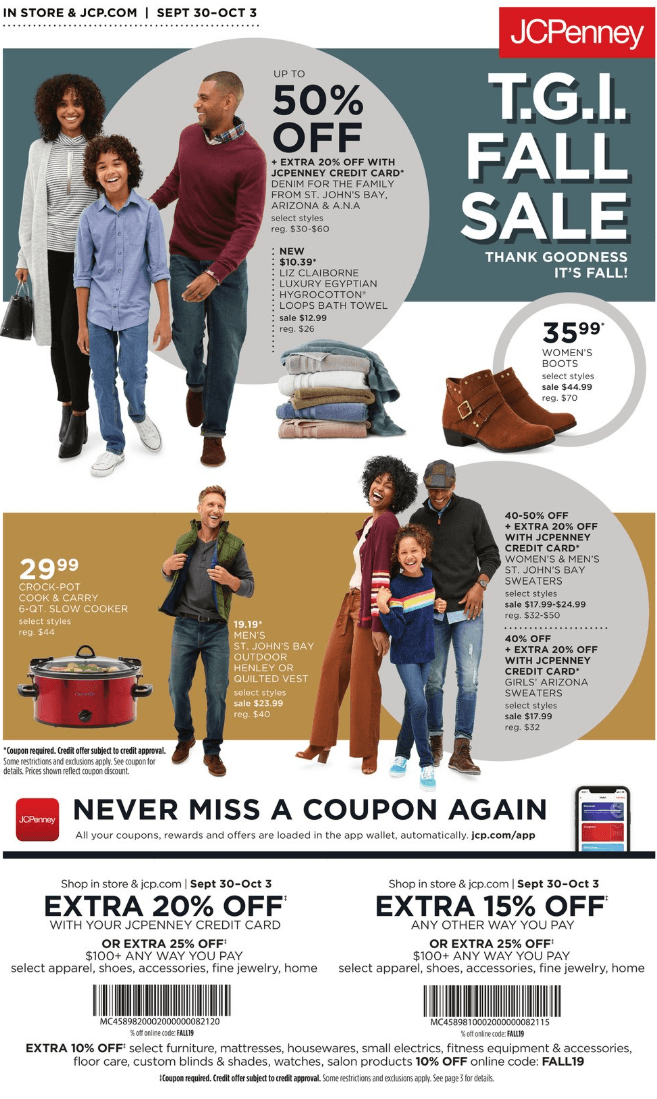This image is a detailed advertising page from the J.C. Penney catalog, prominently featuring various sale items. In the upper right corner, the recognizable J.C. Penney logo is displayed; a red rectangular shape with white text spelling "J.C. Penney."

The top left corner of the page contains black text that reads "in store in JCP.com," alongside the sale dates "September 30th - October 3rd." The main promotional heading is positioned in the upper portion on a teal-gray rectangular background, with white text announcing "TGI Fall Sale" and the subtext "Thank Goodness It's Fall."

The page showcases several individuals, including two women, two children, and three men, all modeling different products. A variety of items are advertised: a neatly stacked collection of clothing, a pair of brown suede boots, and a red crock-pot. At the bottom of the page, there are additional deals highlighted with black text on white backgrounds, consisting of coupons for extra discounts—one offering an extra 20% off and the other providing an extra 15% off. This meticulously arranged page aims to attract customers with a wide array of fall-themed promotions and significant savings.